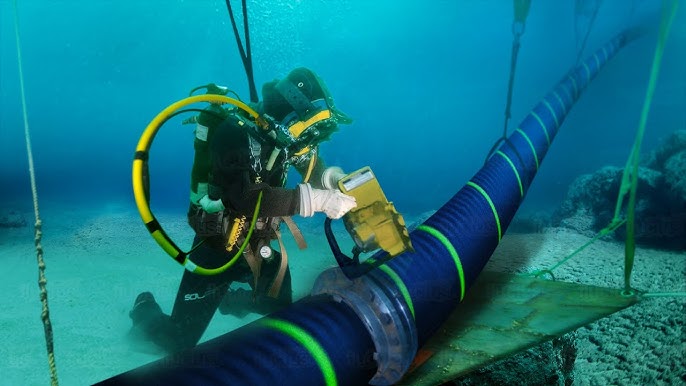In this color landscape photograph, a scuba diver is captured working diligently on the ocean floor. The diver appears to be taking a meter reading from a large blue conduit pipe that stretches diagonally from the top right to the bottom left of the image. The pipe, characterized by its deep blue surface and evenly spaced lime green bands, is suspended from black cables and straps, and secured on a wooden platform with an iron bracket at its center. The diver, who is wearing white gloves, a black wetsuit, and carrying tanks on their back, is kneeling and focused intently on the task, holding a yellow meter instrument pointed toward the pipe. The water surrounding the scene is crystal clear, with sea rocks and sand visible, suggesting that this underwater location might not be excessively deep. The background features a pristine, azure ocean environment devoid of fish, embracing the realism and detail typical of underwater photography in a representational style.